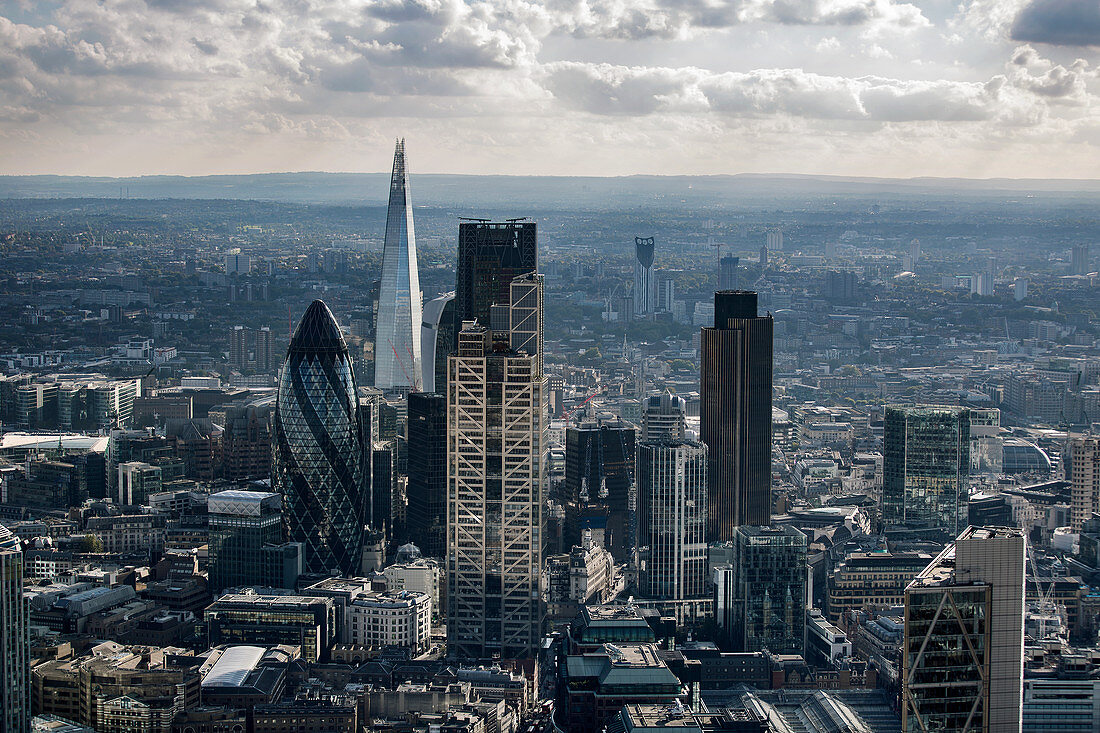This aerial view of a vast, sprawling cityscape captures an impressive scene dominated by modern architecture. The city below is densely packed with a multitude of tall buildings, distinctly devoid of any greenery or trees, emphasizing the urban expanse that stretches as far as the eye can see. The sky above is laden with big, white fluffy clouds, and a gray haze blankets the city, particularly visible in the upper sections of the image, partly obscuring the skyline.

Among the architectural marvels, several iconic and distinctive structures stand out. Most notable is a towering building with a black dome and intricate black swirls cascading down its sides, resembling an ice cream cone with two flavors. This building’s windows are arranged in a spiral pattern, alternating between lighter and darker tones, with the topmost windows completely blacked out. 

To the left of this striking edifice is another significant structure; a skyscraper made entirely of glass with a pronounced, sharp-peaked top and silver hue, reminiscent of a cathedral spire. Adjacent to these is a unique bullet-shaped building with diamond-like silver windows spiraling around its exterior, creating an eye-catching pattern.

Additionally, there is an under-construction building evident from the planking on its side, signaling active development within this immense city. Towards the clearer section of the image center-left, we find a towering hexagon-shaped building made entirely of glass. Overall, this scene is a testament to contemporary urban design, highlighting a blend of functionality and artistic architectural expressions.